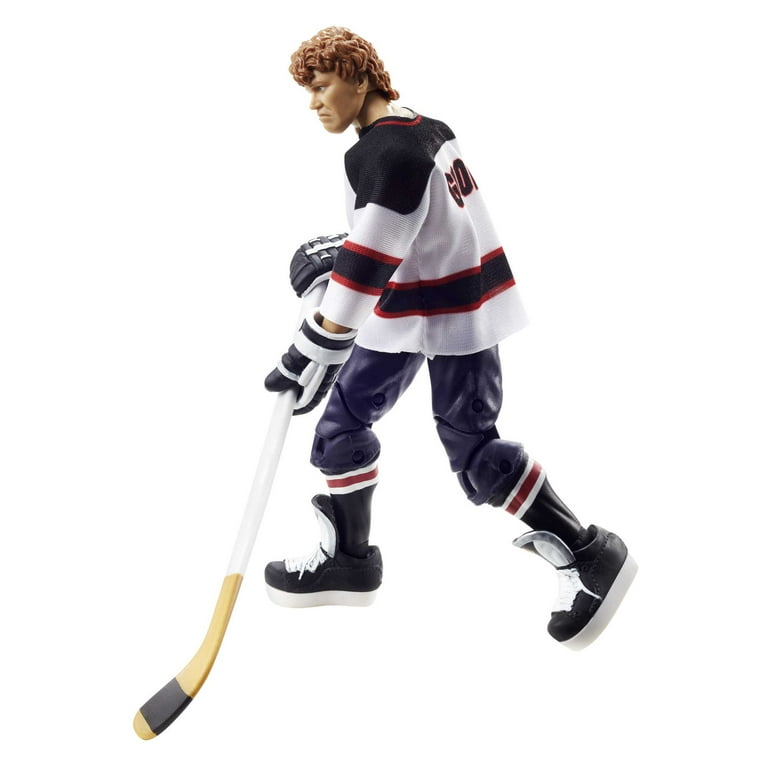This image showcases a toy cutout of a hockey player, standing against a plain white background, likely photographed for a retailer's website. The hockey figurine, approximately 6 to 7 inches tall, features a detailed fabric jersey with black shoulders, a white base, and red and black horizontal stripes, accented with the letters "G" and "O" visible on the back. Sporting light brown, curly hair, the figure gazes off to the left. The player is equipped with large, black and white hockey gloves and holds a meticulously taped hockey stick, painted white with a black band near the bottom. Notably, instead of traditional ice skates, the figure wears sneakers with blue pants and black socks featuring red and white stripes. The majority of the figure, aside from the jersey, appears to be constructed from plastic. The clean white background and absence of additional text or elements keep the focus solely on the uniquely rendered hockey player figurine.